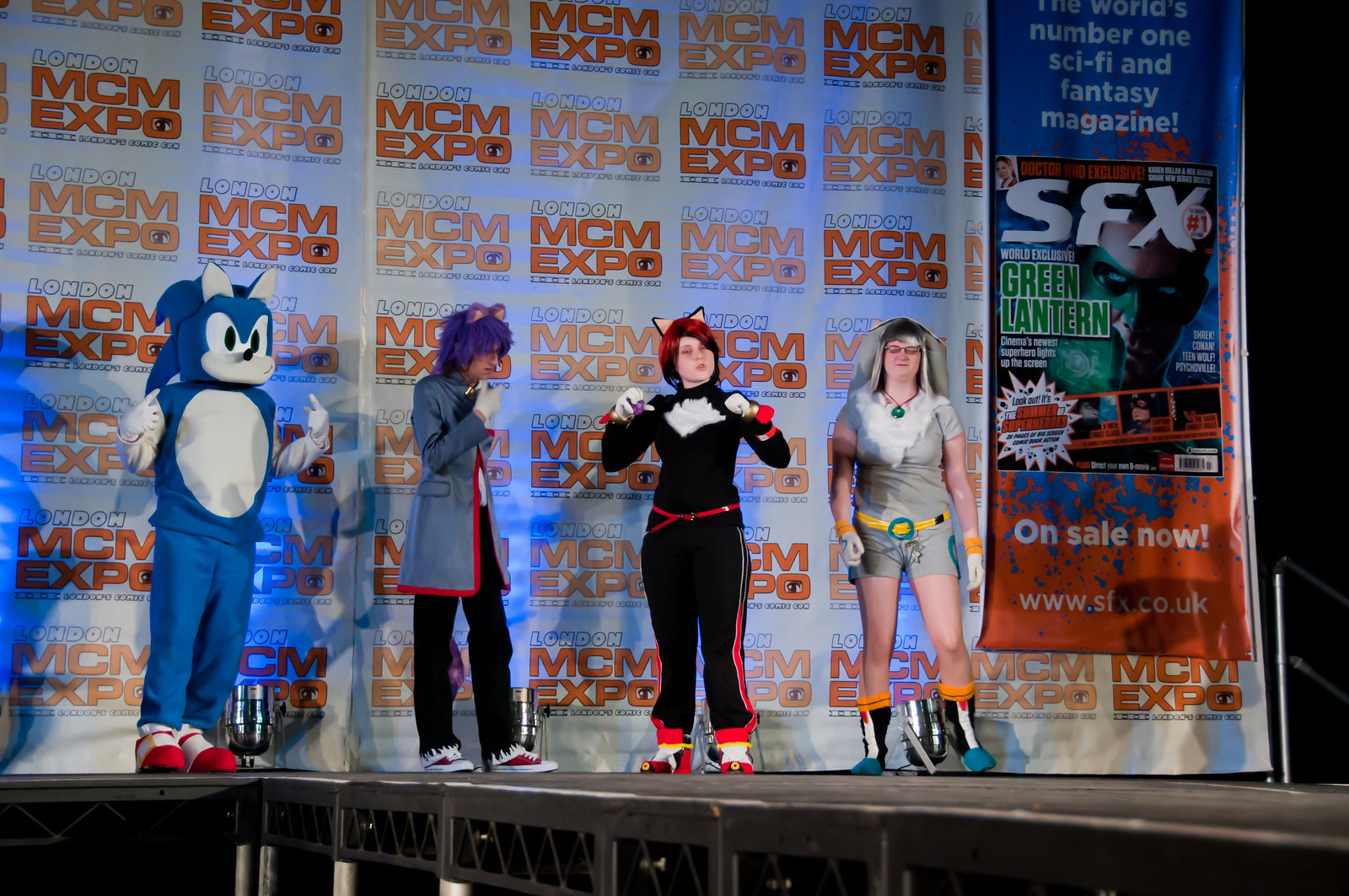In this image, four individuals are performing on a hard-surfaced indoor stage at the MCM Expo in London. Positioned centrally, these individuals are dressed in distinct and elaborate costumes resembling various characters. The backdrop is entirely covered with a repeating pattern of the MCM Expo logo in red letters against a white background.

Starting from the left, the first character appears to be a rabbit-like figure with a white chest and distinct red and white shoes, possibly sporting blue pants. Next to this character is someone with purple hair and rabbit ears, clad in a long gray jacket and black pants. The third character is a woman with red hair adorned with a pink bow, wearing a black outfit featuring a white diamond-shaped design at the top, a red waist belt, and red shoes. The last character on the right is a woman in a silver-colored outfit, which includes short pants and a top. She has silver hair cascading to her shoulders, a green pendant around her neck, and black and white boots.

Additionally, to the right of the stage is a large advertisement banner for SFX magazine, prominently displaying the phrase "number one sci-fi and fantasy magazine" and featuring the Green Lantern along with an "on sale now" note at the banner's orange bottom section. The overall color palette of the image includes black, gray, silver, white, blue, orange, red, yellow, and green, contributing to a vibrant and dynamic scene.